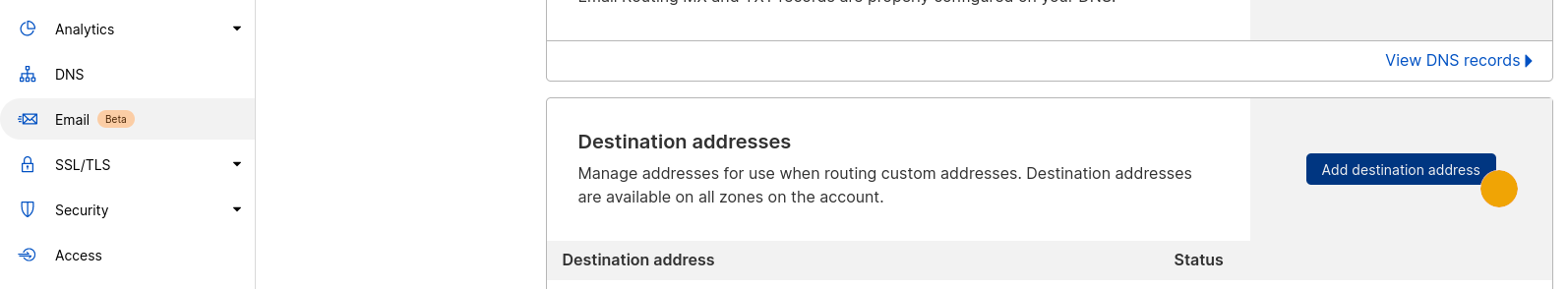The image shows a partial screen capture, primarily featuring a user interface with a white background. On the left side of the image, there is a vertical navigation panel with six menu options listed from top to bottom: Analytics, DNS, Email, SSL/TLS, Security, and Access. The 'Email' option is highlighted with a gray background and has an orange oval labeled 'Beta' next to it.

To the right of this navigation panel, there is some blank space followed by a section displaying parts of two rectangular panels. The top panel is partially cut off. The bottom part of the panel contains a white band with blue text reading "View DNS Records" accompanied by a right-facing caret symbol.

Below this, another rectangular panel spans the width of the screen. This panel has a primarily white background with gray highlights at the bottom and right edges. In the white section, dark gray text reads, "Destination Addresses. Manage addresses for use when routing custom addresses. Destination addresses are available on all zones on the account." To the right within the gray area, a blue button with white text reads "Add Destination Addresses." An orange circle is located at the bottom right of this blue button. Below this, further within the gray section, dark gray text reads "Destination Address" followed by the word "Status" positioned more to the right.